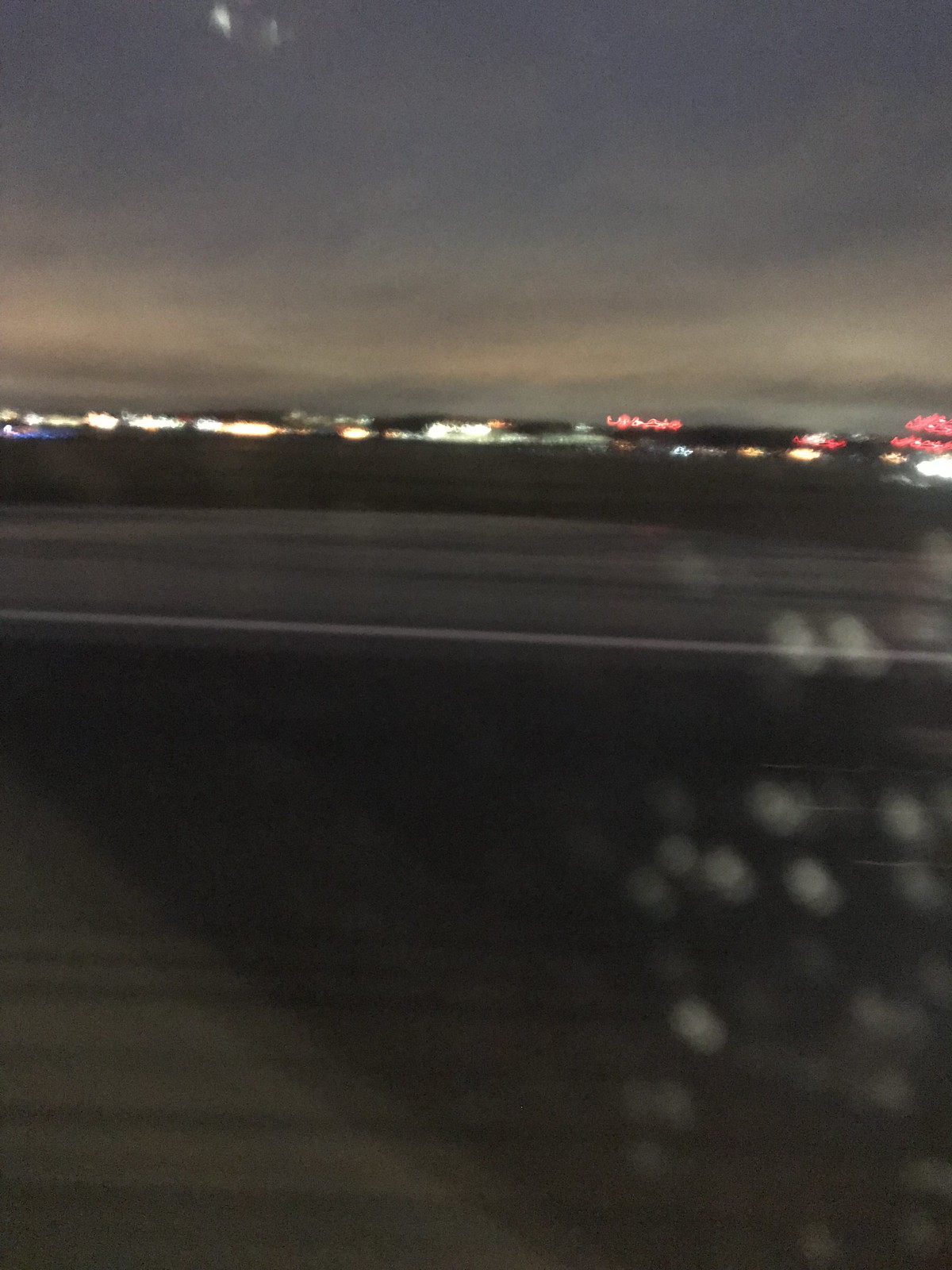The photograph is a blurry, nighttime snapshot taken from inside a car, likely moving. The lower portion of the image is predominantly black with scattered white speckles, possibly reflections or light artifacts. Horizontal light streaks traverse the image, adding to the sense of motion. A slightly tilted white line in the center of the image hints at a road, bordered by a grayish area that merges into another dark section, suggesting distance. Blurry, illuminated spots suggest shops, stores, or buildings in the background. The sky is a gradient from dusky gray to a darker slate gray at the edges, indicating a late evening or early night setting.